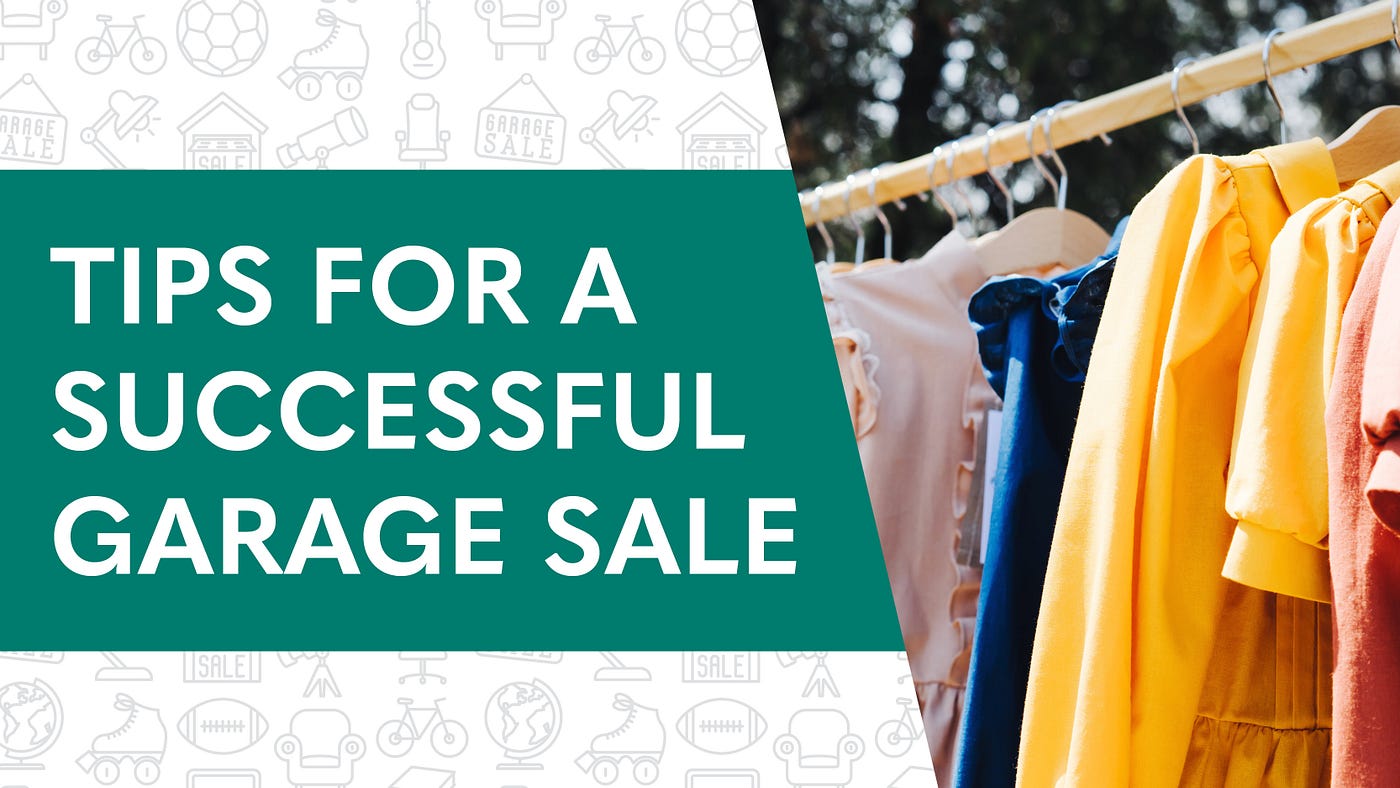This image is a horizontally rectangular advertisement, combining both graphic and photographic elements, likely intended for a blog post about garage sales. The upper left to the center features a light blue background with faint sketches of various items such as bicycles, soccer balls, roller skates, guitars, furniture, football, and a globe. Beneath this area is a teal box with white, all-caps text reading "TIPS FOR A SUCCESSFUL GARAGE SALE." This title is prominently displayed in three lines against the greenish background. The right side of the image showcases a colorful photograph of vibrant female clothing hanging on a white rack, with garments in pink, blue, yellow, and other hues. The rack extends from the green area on the left up to the top right corner, and the clothes drape off the bottom of the image. Above the clothes, a clear blue sky and some trees are visible, indicating that the photograph was taken outdoors during the day. The combination of these elements creates a vivid and informative visual intended to draw attention to tips for organizing a successful garage sale.